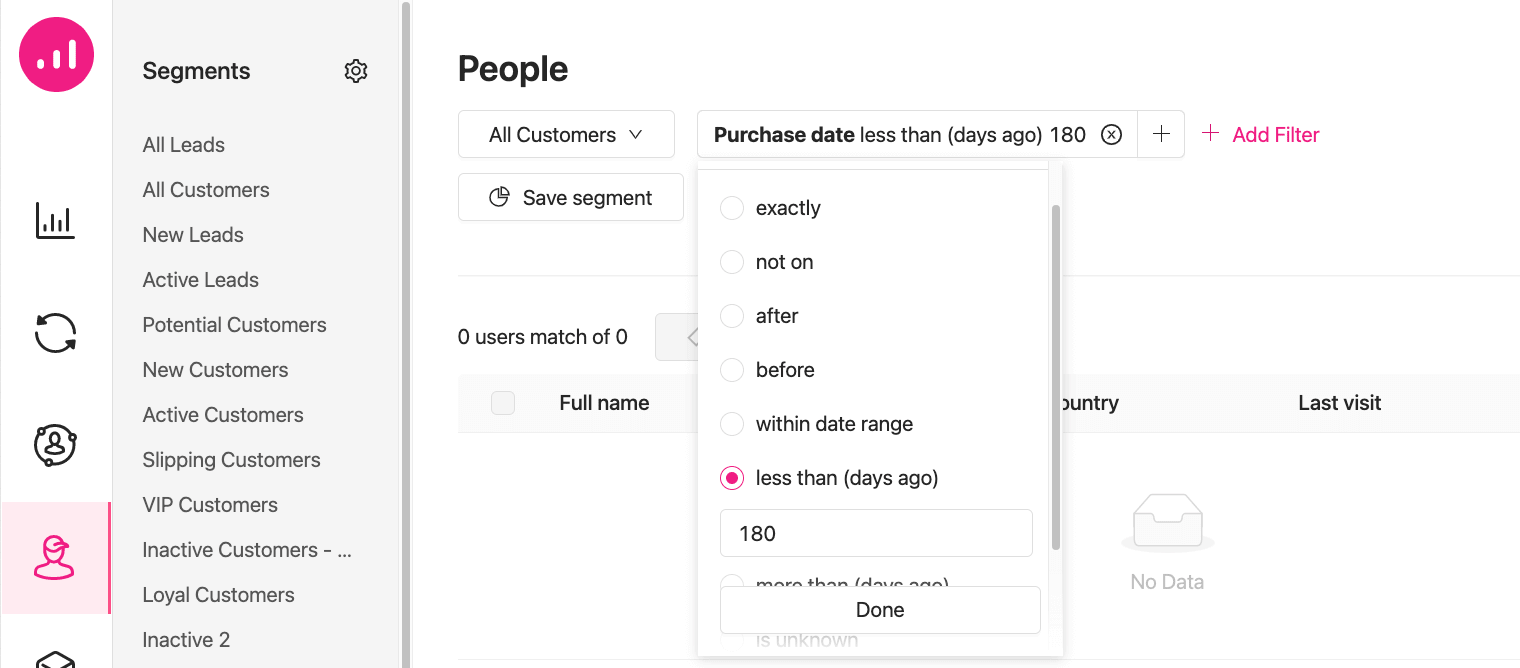The image displays a dashboard with a variety of icons and filters on the left-hand side. At the top, there's a gray vertical line dividing the interface. The first icon is a bar graph within a pink circle, indicating it is in focus. Below it, there are three staggered horizontal lines of increasing length. Following this, there is another bar graph, not in focus. 

Next, there's a circular icon with two arrowheads forming a loop, resembling a rounded arrow. Down further is an icon depicting a person inside a dotted circle. Adjacent to this, there's another person icon, this time with a baseball cap inside a pink box, which is highlighted, indicating focus. Partially visible below these icons is another cut-off icon.

Moving to the right, there's a "Segments" section featuring a gear icon for settings. The section lists several categories in bold black text, including All Leads, All Customers, New Leads, Active Leads, Potential Customers, New Customers, Active Customers, Slipping Customers, VIP Customers, Inactive Customers, Loyal Customers, and Inactive too, with a toolbar to scroll through more options. Below this, the title "People" appears alongside a dropdown menu labeled "All Customers" and a filter box labeled "Purchase Date Less Than 180 Days Ago," next to an X in a circle and a small square with a plus sign inside.

Further down, a button labeled "Add Filter" is displayed in pink text with a pink plus sign. The "Save Segment" button is situated directly below this. Radio buttons are available with options such as "Exactly," "Not On," "After," "Before," "Within Date Range," and "Less Than 180 Days Ago," with "Less Than" in focus, highlighted by a pink radio button. Below these, additional options include "More Than" and "Unknown," paired with a "Done" button that remains unclicked.

Behind this active area, a partially obscured section features phrases like "Zero Users," "Match of Zero," and "Full Name" next to text boxes, along with a "No Data" box at the bottom, making it difficult to determine the purpose of these elements due to overlapped content.